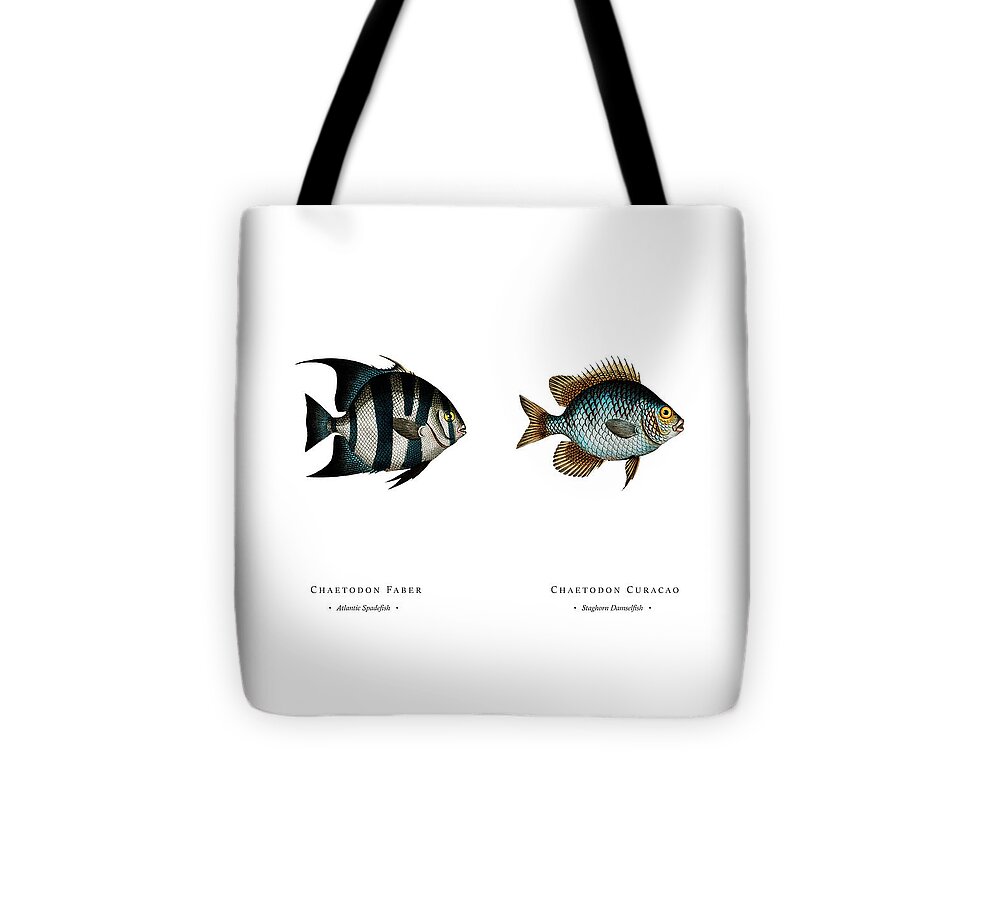The image features a white tote bag against a white background. The bag itself is shaped like a vertical rectangle and is adorned with two black straps attached to its top corners. On the front of the tote bag, there are two horizontally placed fish, centered in the design. 

The fish on the left, labeled "Chaetodon Faber," displays a gray body with vertical black stripes and dark blue fins, and is shaped like an oval. Below its name, "Atlantic Spadefish" is written in black text. To the right, a fish labeled "Chaetodon Craco" exhibits light blue coloring with a dark blue top, along with dark brown fins. Text beneath it also includes the scientific name "Chaetodon" in black. The detailed representation of the fish, along with their names, makes the design both informative and visually appealing.